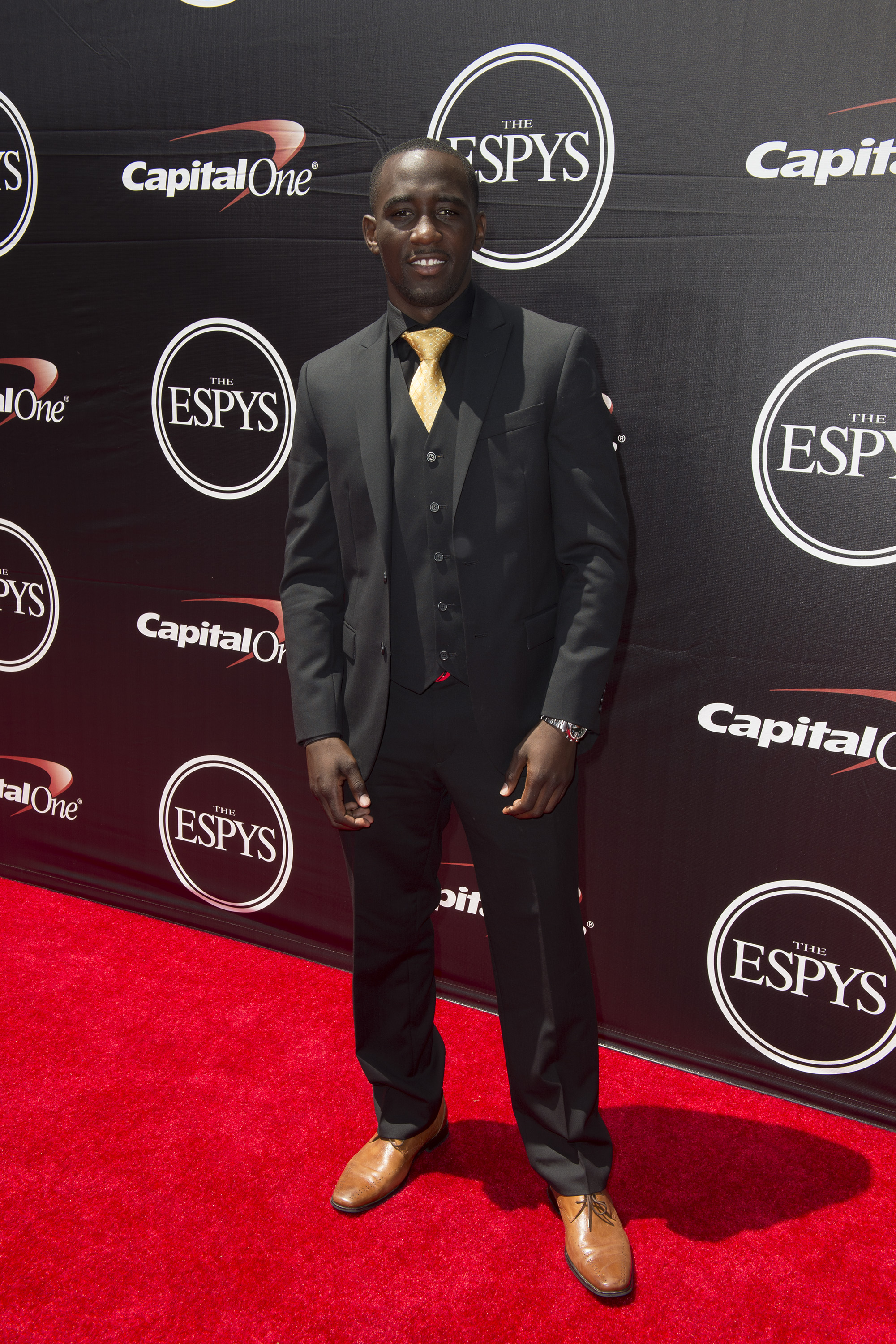In this photograph, an African American man stands confidently on a red carpet. He is dressed impeccably in a black suit, featuring a black coat, vest, and pants, paired elegantly with a golden-colored tie and brown shoes. His silver watch peeks out from his left wrist. The man exudes a subtle charm with his short black hair, slightly open mouth forming a half-smile, and white teeth. He stands in front of a black step-and-repeat banner adorned with various logos, including Capital One in a white circle with a distinctive red boomerang shape, and repeated ESPYs logos encased in white double circles bisected by a black line. His full-length body is visible, with his hands resting near his hips, facing slightly towards the right, casting a shadow on the red-carpeted ground.